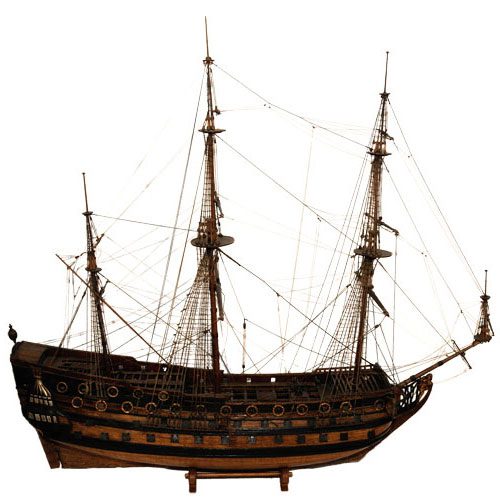This detailed photograph features a meticulously crafted model of a three-masted sailing ship, reminiscent of the 1700s-1800s era, often associated with vessels like those of Christopher Columbus. The model, set on a small wooden stand, is captured against a stark white background, putting the ship's intricate details into sharp focus. The dark and lighter brown hues of the wooden boat contrast with the meticulously interconnected rigging that spans between the three towering masts, which lack sails. The masts, featuring multiple platforms of varying sizes and ladders, highlight the ship's complex rigging system. The mast nearest the stern has a smaller platform and two further reduced levels above it, while the second and third masts have larger platforms and even reach a fourth level at the top. Lines of ropes and wires crisscross between these structural supports. The ship also showcases several life preservers along its sides, and a stick-like bowsprit extends forward with a triangular element mounted atop it. Further adding to the ship’s authenticity, portholes and rectangular windows line the vessel’s sides, accented by a distinctive black stripe near the hull. The image is taken from a slight overhead perspective, providing a view of both the side and part of the top deck, enhancing the historical richness and maritime intricacy of the model.